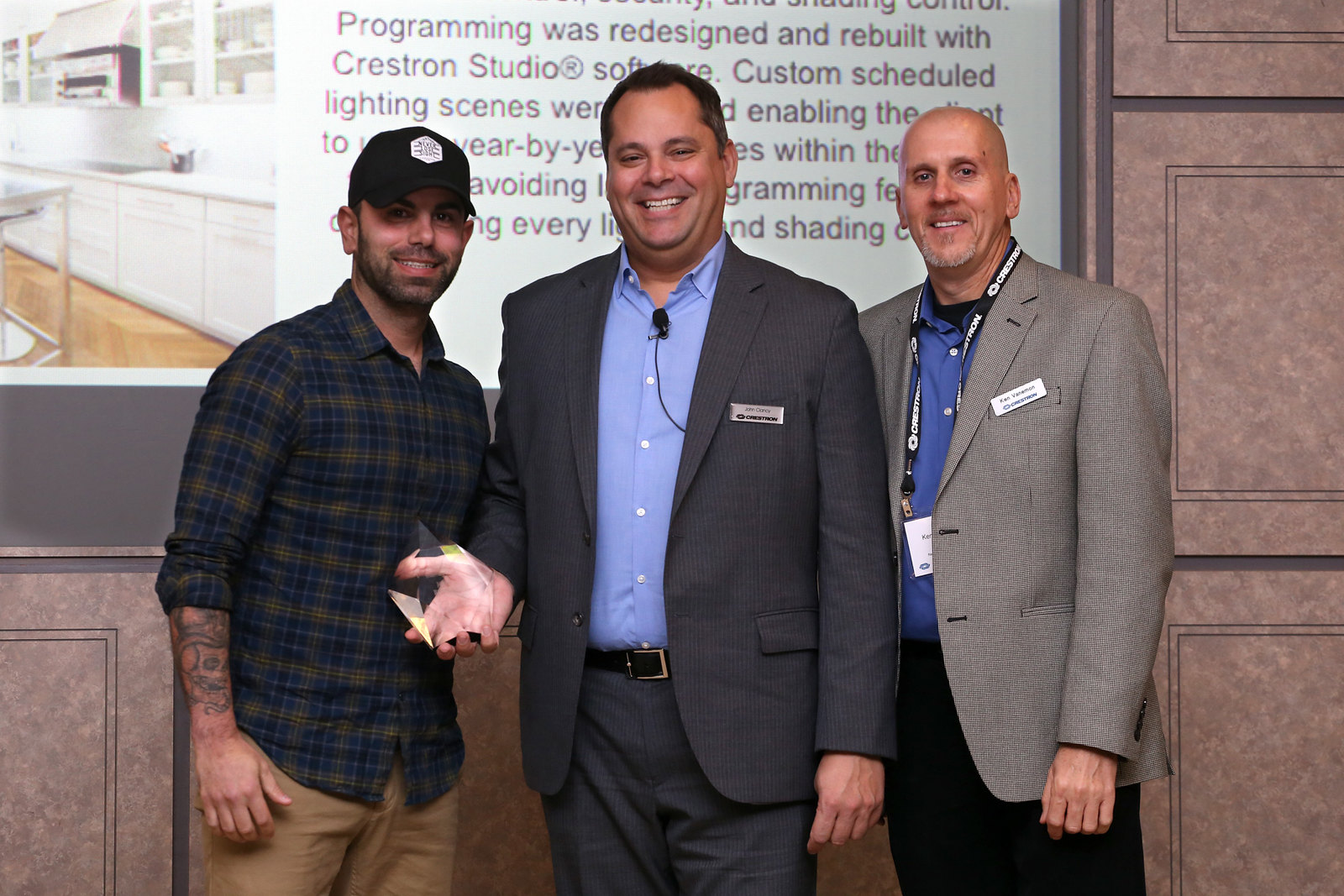In this photograph, three men are standing close together, posing for a picture and smiling at the camera. They are positioned in front of a wall covered with brown square tiles and featuring a large, visually prominent poster. The poster has a detailed image of a kitchen along with some text on a white background, which reads, "programming was redesigned and rebuilt with Creston Studios software, custom scheduled lighting scenes," although the rest of the text is obscured by the men.

On the left is a younger man wearing a black baseball cap, a plaid shirt in shades of blue and green, khaki pants, and he has a tattoo on one of his arms. In the middle stands an older man dressed in a gray pinstripe suit with a light blue dress shirt. He is holding a clear, glass award in his hands, which is intricately shaped and molded. To the right is a bald man sporting a light gray suit jacket, a darker blue collared shirt, black pants, and a lanyard around his neck. The photo captures the men's faces, upper bodies, and legs up to their knees.